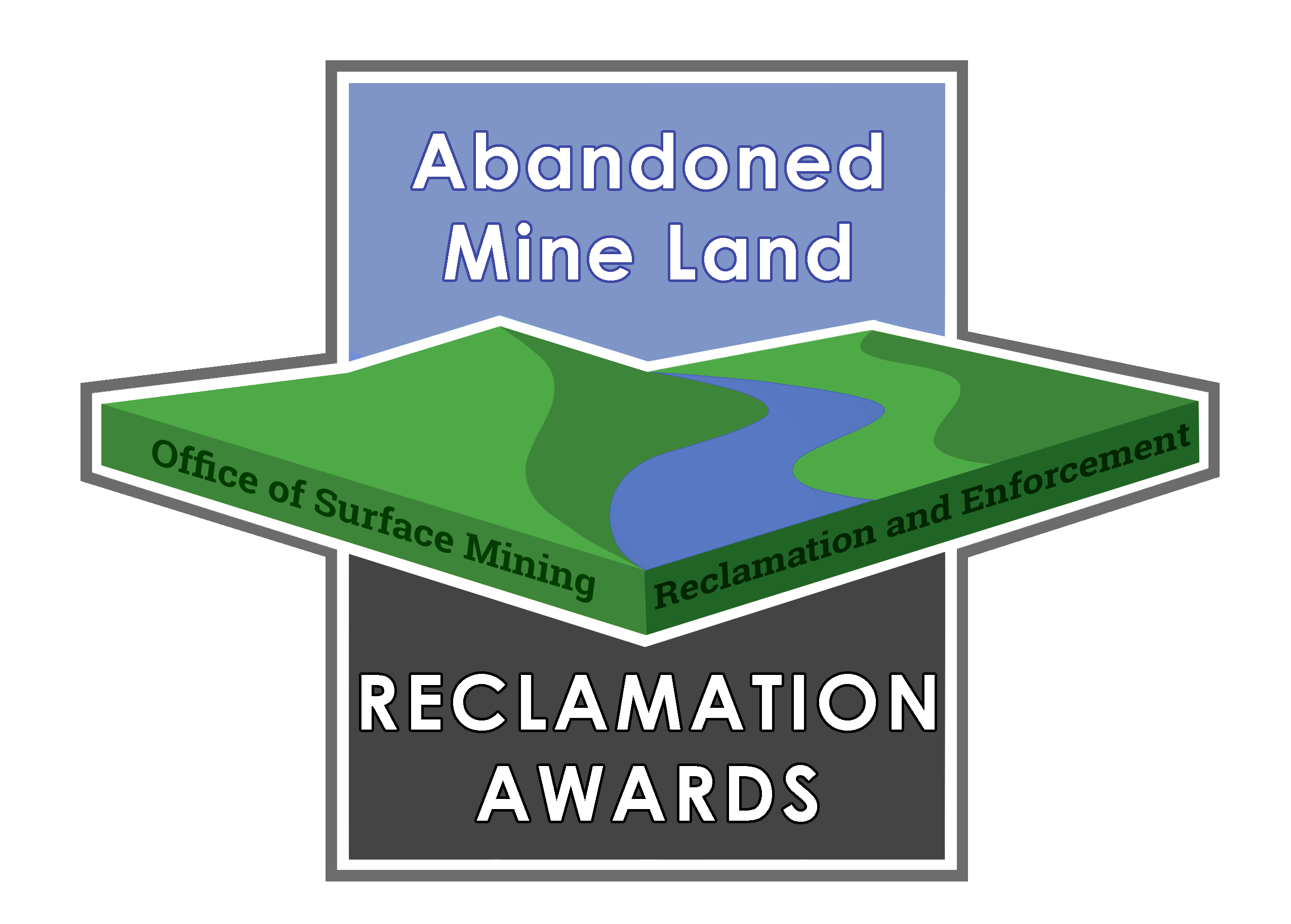The image depicts a detailed logo for an award, specifically the Reclamation Awards presented by the Office of Surface Mining, Reclamation, and Enforcement related to Abandoned Mine Land. The logo is primarily a vertically oriented rectangle divided into two halves: the top half features a light bluish-purplish background with the text "Abandoned Mine Land," and the bottom half has a dark gray background with the text "Reclamation Awards." In the center of the rectangle, there is a prominent 3D diamond shape projecting out, with one of its points directed towards the viewer. The diamond is designed to resemble terrain, with green hues representing land and a blue river running through it. The diamond also bears the text "Office of Surface Mining, Reclamation, and Enforcement" along its sides. The overall design uses a white outline to highlight the 3D effect, creating the impression of a model rather than a real landscape. The letters within the logo are bold and vary in color, enhancing the visual impact.